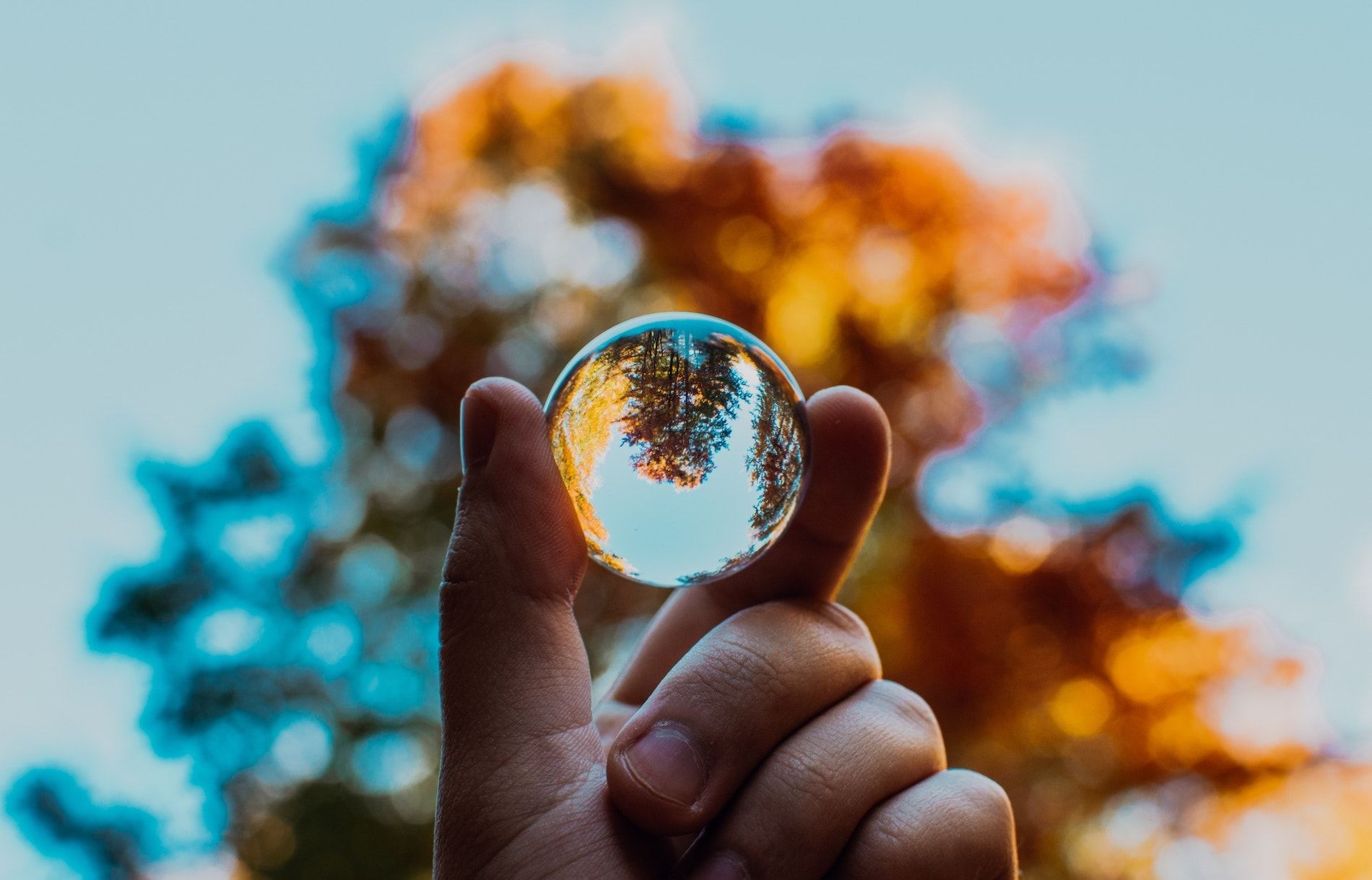The image is a close-up photograph of a person's left hand holding a small glass sphere between their thumb and index finger. The person's nails are cut very short, displaying the pink of their fingertips. Inside the fragile glass sphere, there is a captivating reflection; at the top of the sphere, an upside-down tree is prominent against a blue sky, while a hint of light yellow sun and green foliage color the reflection. The actual background of the photo is blurred, but it matches the reflected scene with a light blue sky and the seasonal hues of the tree, rendering the overall image both intricate and strikingly vivid.